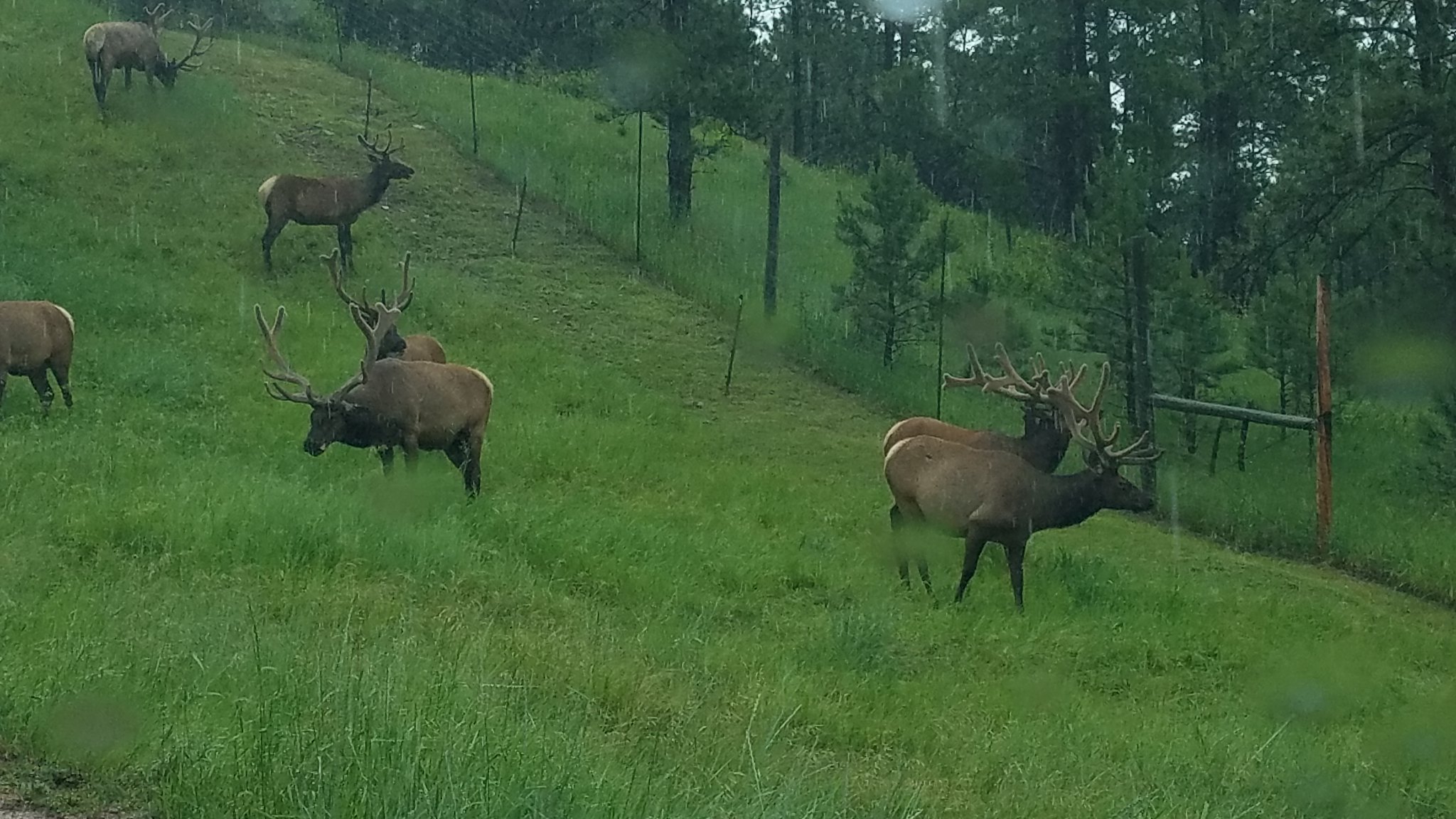The photo captures a vibrant emerald green meadow with a variety of elements that create a serene yet lively scene. Dominating the meadow are six or seven large, mature moose, distinguished by their impressive, thick antlers which are a tan color and intricately branched. Their fur is a mix of dark brown and light tan, with the darker shade covering their head, neck, legs, and lower stomach, while their back and butt are of a lighter tan hue. Some of these majestic animals are grazing on the long, sharp blades of grass, while a couple of them look over a barbed wire fence supported by brown posts, which trails up the sloping hill.

In the background, a dense forest of evergreens stretches across the horizon, their deep green leaves contrasting with the bright meadow. The scattered rays of the morning sun peek through the foliage, casting dappled light across the scene and indicating that it is indeed daytime. The overall composition paints a detailed and serene picture of wildlife in its natural habitat, perfectly captured on a crisp morning.